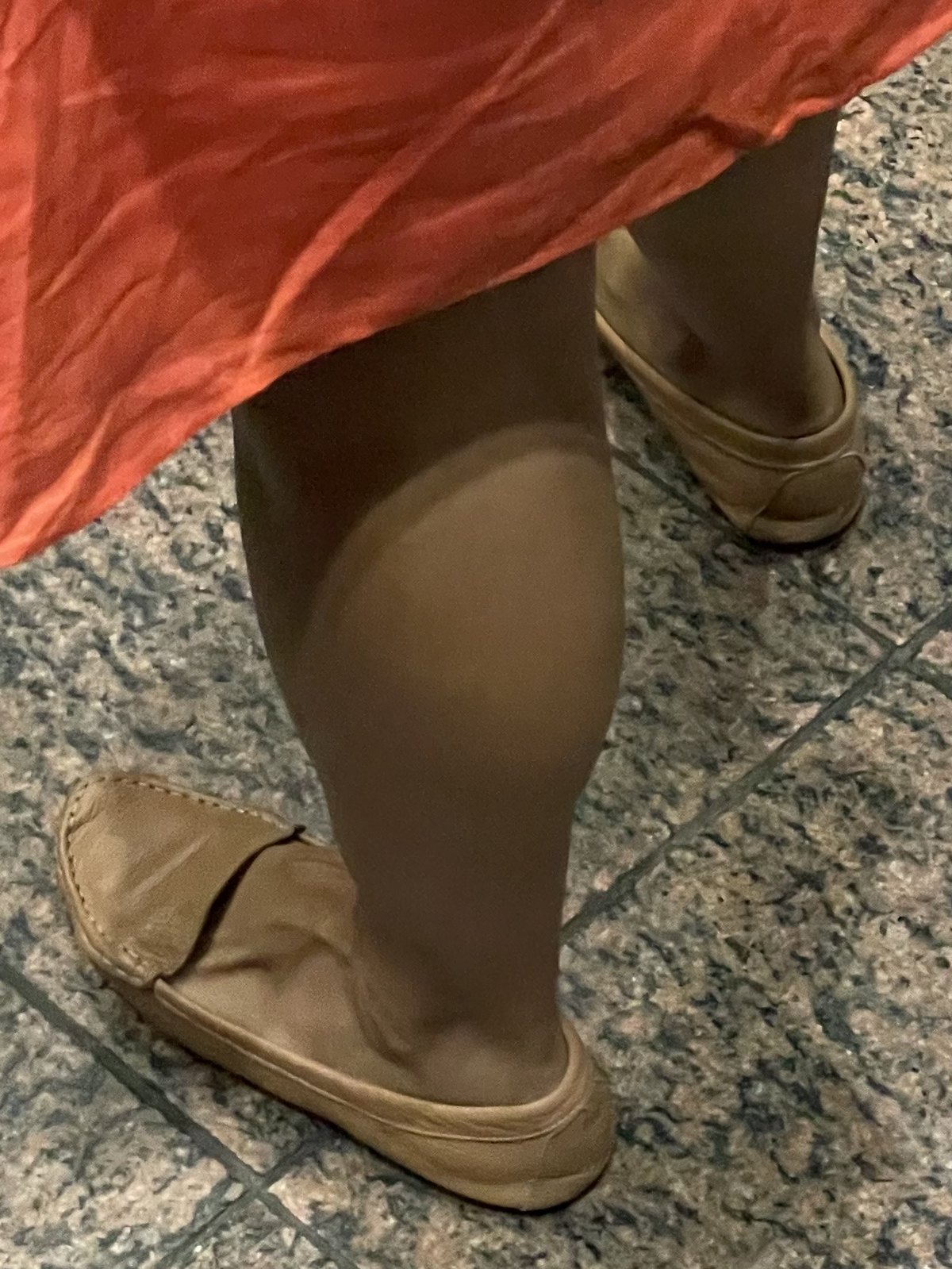This image is an extreme close-up of an African-American woman's legs and feet, viewed from a top-down angle. Her smooth, defined calf muscles suggest she is possibly an athlete. She is wearing brown slip-on shoes that blend seamlessly with her tan skin tone. The woman is clad in a red fabric, which could be a skirt, a dress, or even a shawl, visible up to her calves. She stands on a tiled floor that features a mix of reddish-gray, black, and brown hues, likely in an office building. The overall composition focuses on the legs, the red fabric, and the distinctively patterned tile floor.